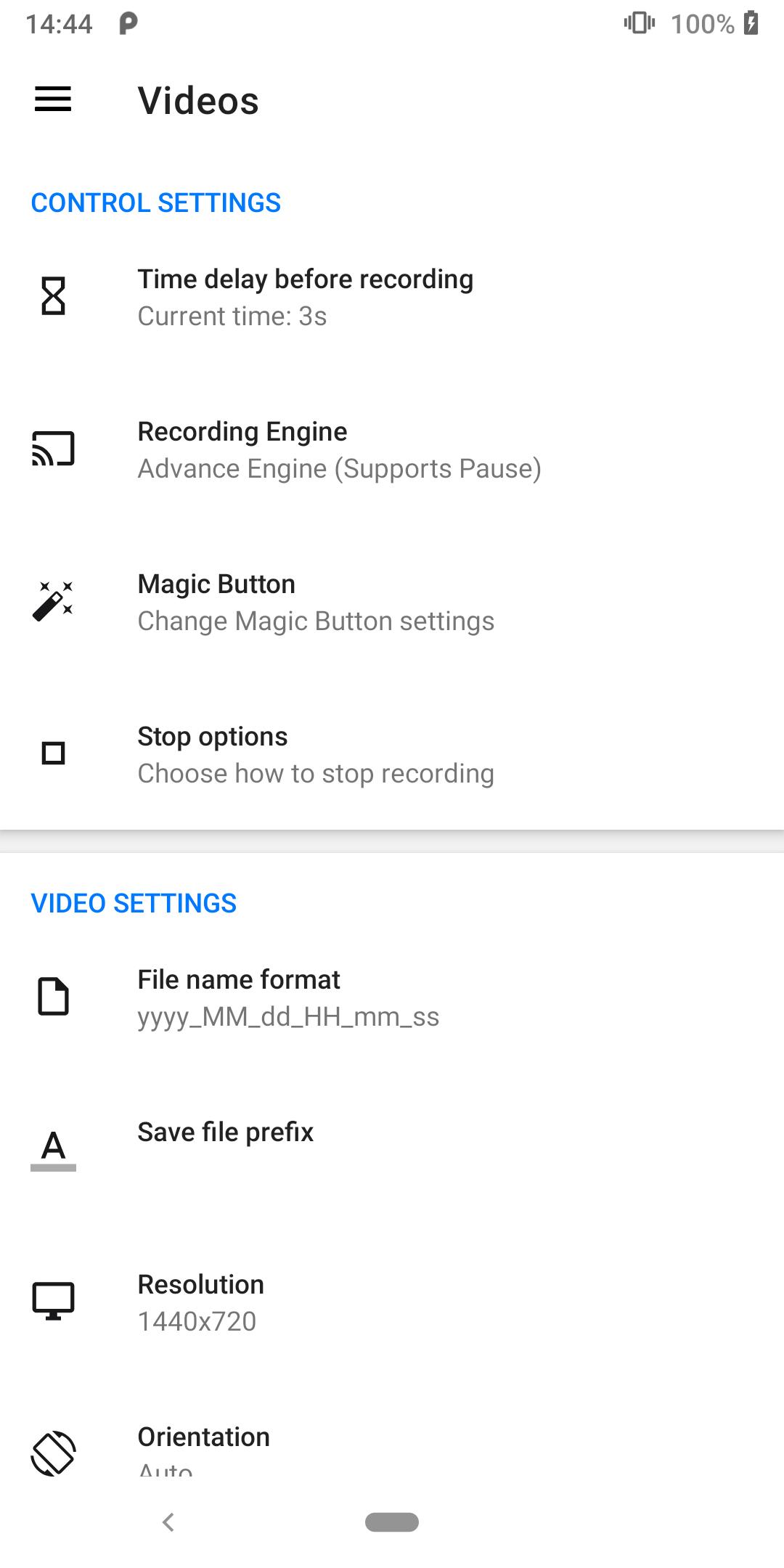This image is a screenshot from a cell phone, featuring a plain white backdrop. About halfway down the screen, a light gray horizontal border approximately a quarter of an inch wide runs across from left to right. In the upper left corner, the time "14:44" is displayed, next to a bold letter "P". The right side of the screen shows a battery icon at 100% and a vibrate mode icon to its left.

Beneath the time display "14:44" on the left, three parallel black lines each about a quarter-inch long are stacked one above the other. To their right, the word "Videos" is displayed in normal font, followed by a small space, and then "CONTROL SETTINGS" in blue, all capital letters.

The lower section of the screen is divided into two main parts by the aforementioned light gray border. 

Above the border, on the left side, four icons are listed vertically, each accompanied by descriptive text to its right. The first icon is an hourglass, labeled "Time of delay before recording" in black. Below this, in grayish-black text, it reads "Current time: 3 seconds." This pattern continues with three more icons, each with corresponding descriptive text.

Below the light gray border, the section is labeled "VIDEO SETTINGS" in blue text. Below this heading, there are four more icons listed vertically on the left, each accompanied by bold black text to the right, and additional descriptive grayish text beneath it. The first icon appears as a piece of paper with a folded upper-right corner, labeled "File name: fortnite" in bold black text. Underneath, in gray, it reads "yyyy_mm_dd_hh_mm_ss." This structure replicates for three additional icons with varying information.

Centered at the very bottom of the screen, there is a small gray bar about half an inch long. The detailed structure and compact information suggest a sophisticated settings interface for a video recording application.